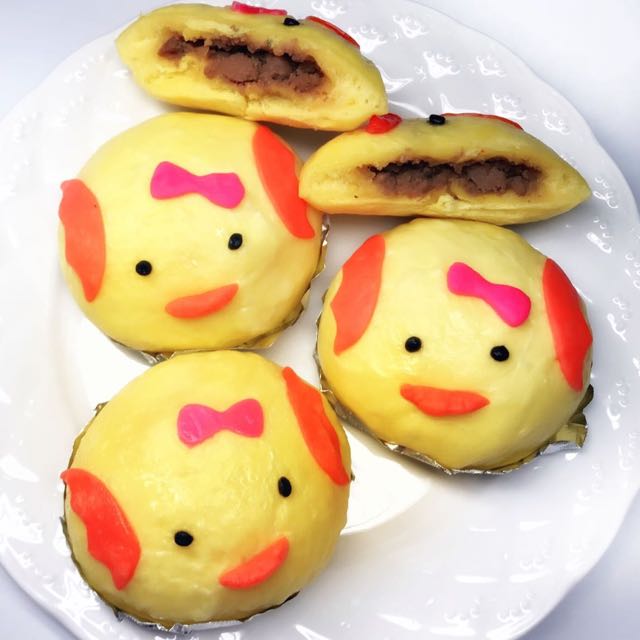The photograph showcases four charming yellow bao buns meticulously arranged on a shiny round white plate against a plain white background. Each bun is adorned to resemble a little chick, complete with small black eyes, an orange beak, and orange wings on either side. Adding a touch of whimsy, each chick sports a pink bow on top. The buns are nestled in individual silver tinfoil cups. Notably, the fourth bun at the back is cut in half, revealing a chunky brown filling inside.